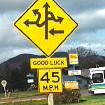The image depicts a humorous road sign intended to resemble a cautionary warning but with an added twist. The sign is triangular, though the top part is cut off. The background color is yellow with a black border, giving it an authoritative appearance. Centered on the sign is a set of multiple, confusing arrows: one arrow points straight up, another points to the left, a third diagonally up and to the left, a fourth points to the right, and an additional arrow is attached to the diagonal left arrow, pointing left as well. Beneath this chaotic array, the words "GOOD LUCK" are boldly capitalized. The sign also indicates a speed limit of 45 miles per hour (mph). The overall effect suggests a humorous commentary on confusing road directions, leaving drivers with a cheeky "good luck" message to navigate the impending complexity.